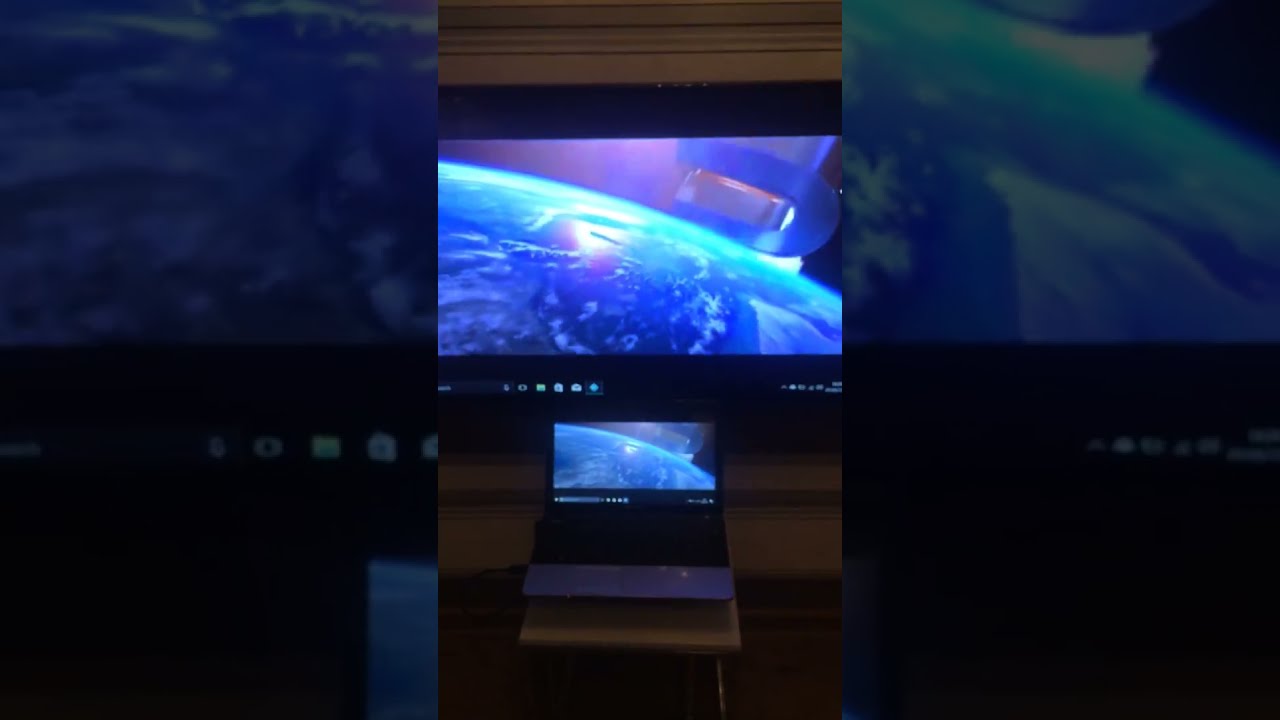The image captures a scene with a laptop positioned on a brown, striped tabletop, set within a primarily dark environment. The laptop, featuring a standard 15-inch screen, displays a dynamic, colorful visual dominated by hues of blue, orange, and white lights. The on-screen content suggests a high-speed movie scene, possibly a car chase, characterized by bright circular lights and vivid streaks of color. This same visual is mirrored on a significantly larger TV screen, possibly between 50 to 55 inches, located directly in front of the laptop. The image feels slightly blurred and in motion, enhancing the impression of high-speed action. Notably, there are no visible cables, implying the devices might be connected wirelessly, potentially via Bluetooth. The sides of the image include simple black borders, isolating the central focus on the vibrant screens within what could be a dark classroom or a home setting.